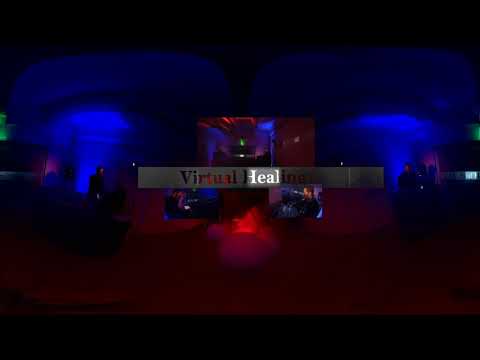The image depicts a dark, likely indoor stage scene with dramatic lighting and a smoky atmosphere, suggesting a concert or performance setting. Dominating the center, there's a blotch of fluorescent red light shrouded in darker red light, reminiscent of smoke, which casts an ethereal glow over the scene. A prominent gray banner hangs in the center, displaying the partially lit words "Virtual Heal" - with "heal" illuminated more brightly than "virtual." The red background can be seen through some of the letters. Flanking the top left and right corners are blue fluorescent lights that transition from white at the center to darker hues, ultimately fading into the black background. On the right, a silhouetted figure stands against the blue light. Additional figures, possibly band members with instruments, are faintly visible on stage, contributing to the impression of a live musical performance amidst dynamic red, blue, and occasional green lighting effects. Enclosed within a black frame, the overall aesthetic hints at either a technologically themed event or an immersive stage show, possibly tied to a "Virtual Healing" narrative.